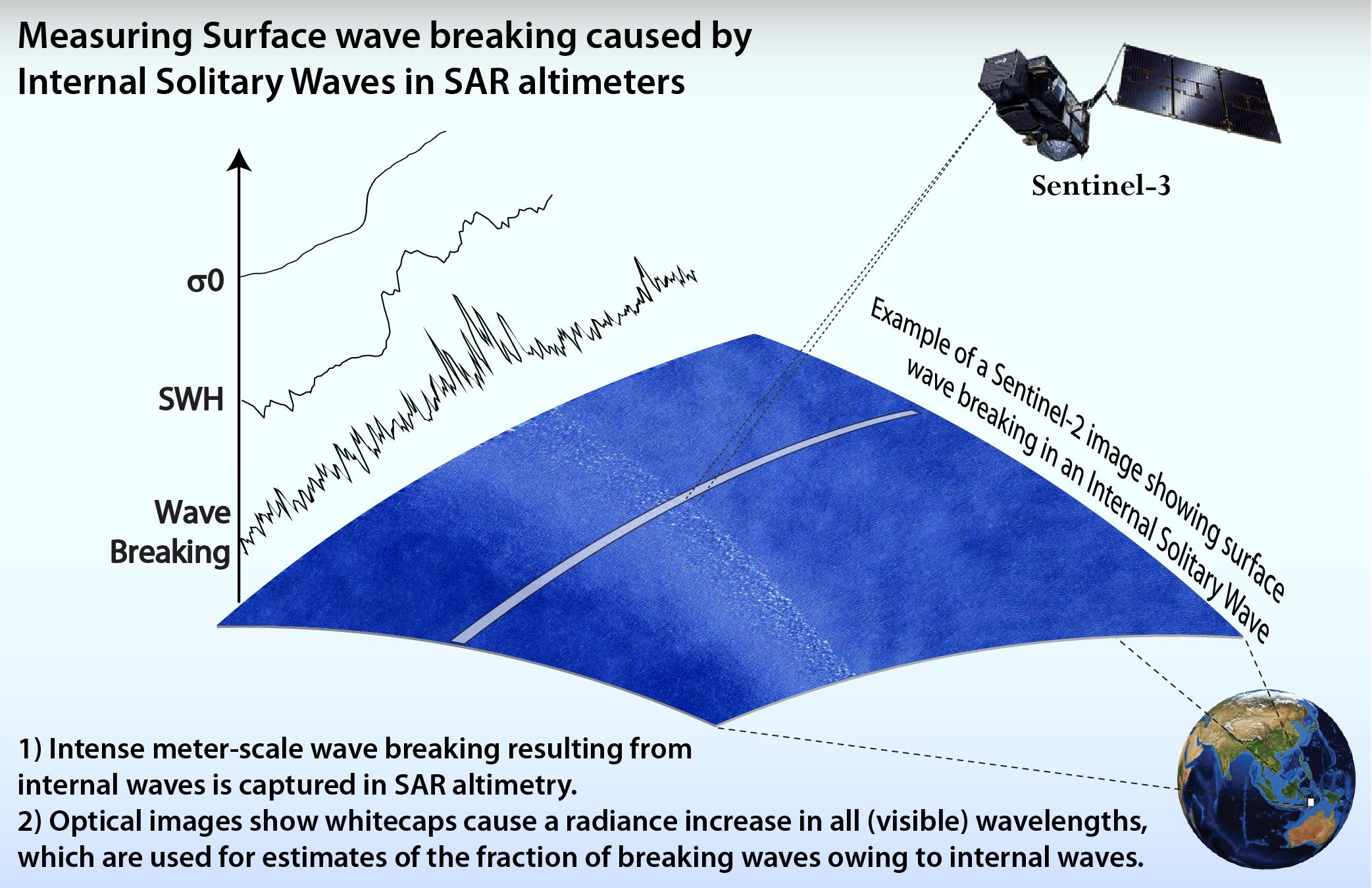The image is a detailed scientific diagram titled "Measuring Surface Wave Breaking Caused by Internal Solitary Waves in SAR Altimeter." It includes multiple elements that illustrate the phenomenon.

At the center of the image, there's a warped, diamond-shaped graph in dark blue, representing data collected by SAR altimetry. The graph has an arrow pointing upward labeled "wave break," with sections marked SWH (Significant Wave Height) and another scientific symbol, each accompanied by waveform illustrations indicating progression.

To the top left, there is a title highlighting the study on surface wave breaking, while the top right features an illustration of a small, boxy satellite equipped with a solar panel, identified as Sentinel-3. Below the satellite, in black text, it reads, "example of Sentinel-2 images showing surface wave breaking in an internal solitary wave."

The bottom right section displays a circular depiction of the Earth, with colors blending from dark and light blue to brown and green, against a background that transitions from white at the top to light blue at the bottom.

Additionally, the bottom left contains annotations with detailed observations: 
1. "Intense meter-scale wave breaking results from internal waves is captured in SAR altimetry."
2. "Optical images show white caps causing a radiance increase in all visible wavelengths, which are used for estimates of the fraction of breaking waves owing to internal waves."

This detailed composition, likely from an educational textbook, efficiently illustrates the correlation between SAR altimeter data and optical imagery in studying internal solitary wave-induced surface wave breaking.